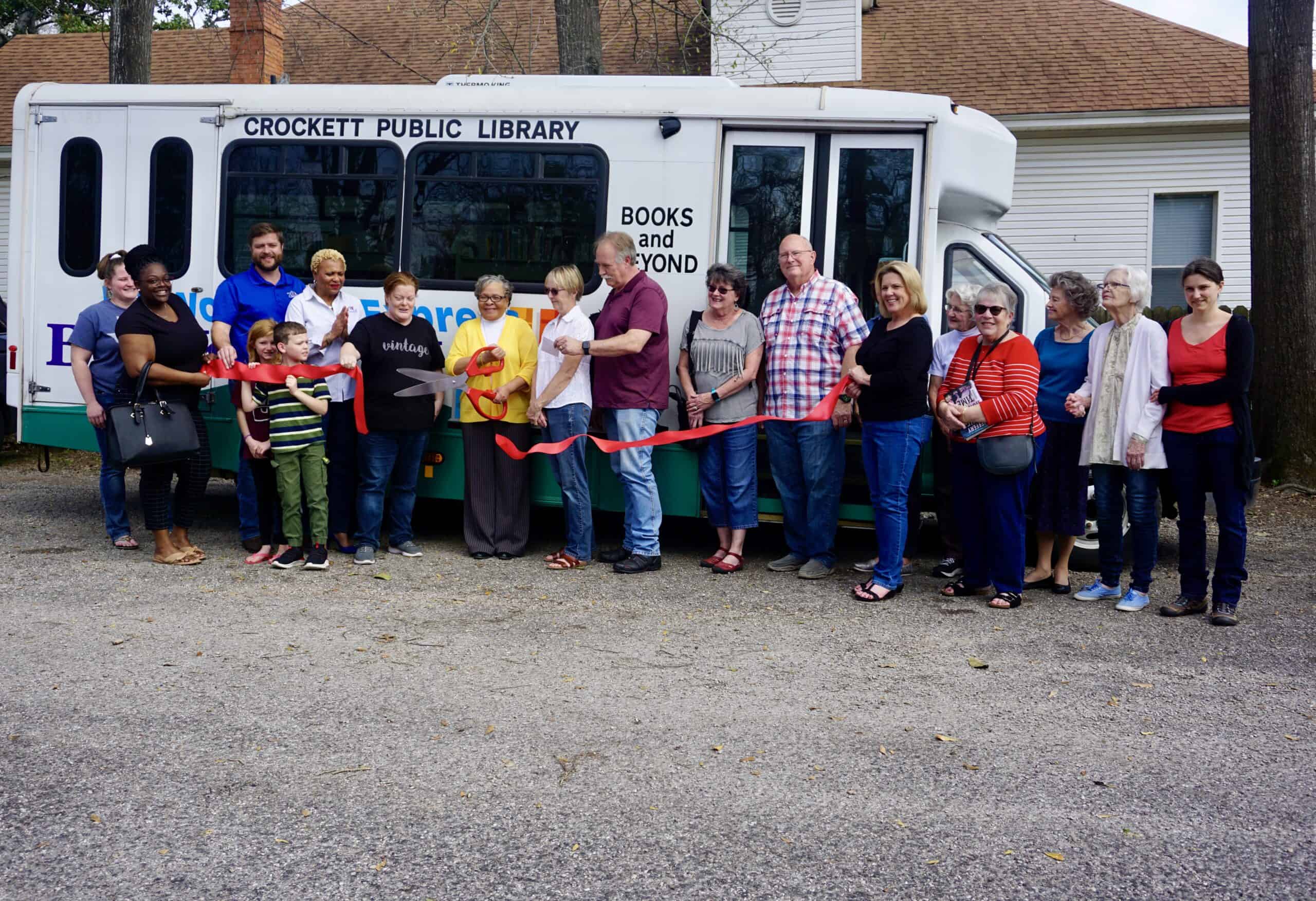A diverse group of community members, ranging in age from young children to elderly adults, is gathered for a celebratory ribbon-cutting ceremony in front of a white bus with a green trim. The prominently displayed text on the bus reads "Crockett Public Library" and "Books and Beyond." This specially equipped bus, featuring wheelchair-accessible doors, stands in front of what seems to be an older, established library building. The red ribbon that has just been cut with a pair of large scissors placed slightly left of center, symbolizes the inauguration of this mobile library service aimed at improving access to the library's resources for everyone in the community. Approximately 10 to 15 people, dressed in a variety of colors and patterns, exude excitement and happiness despite the overcast weather, as they either prepare to board the new service or are simply celebrating the achievement.